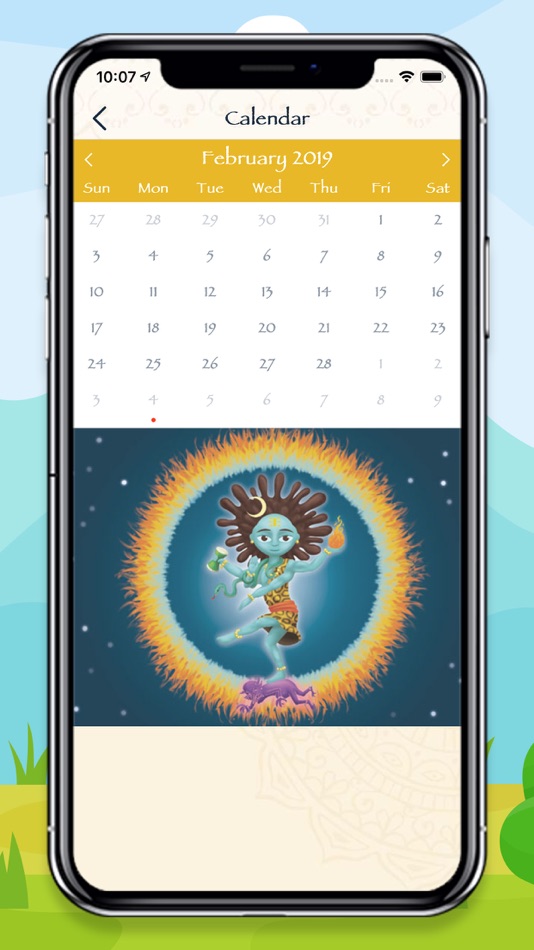The image features a sleek cell phone against a vibrant, cartoon-style backdrop. The background showcases a lush grassy area at the bottom, complete with tufts of green grass and a bush on the right side. Above the greenery, a series of mountains in varying shades of blue rise towards a sky filled with clouds in different hues of white and blue, all under a small patch of light blue sky at the top.

Prominently placed in front of this scenic background is a cell phone with a shiny black bezel and rounded corners. The phone's left side has several silver buttons, mirrored by one button on the right. At the top and center of the phone, a small black rectangular area with rounded corners stands out. 

Displayed on the phone's screen is a calendar and an image. The calendar’s header is in a rich mustard yellow or orange hue with "February 2019" written in a crisp white font, flanked by white left and right arrows. Days of the week are listed in white as Sun, Mon, Tue, Wed, Thu, Fri, and Sat, followed by the dates 1 through 28 in a darker shade, contrasting with the lighter dates from the previous and following months. Notably, this month starts on a Friday.

Below the calendar, there is a cartoon-style illustration of a Hindu god, set against a deep blue background adorned with scattered stars. This detailed composition combines a modern technological interface with traditional cultural elements, providing a rich visual experience.